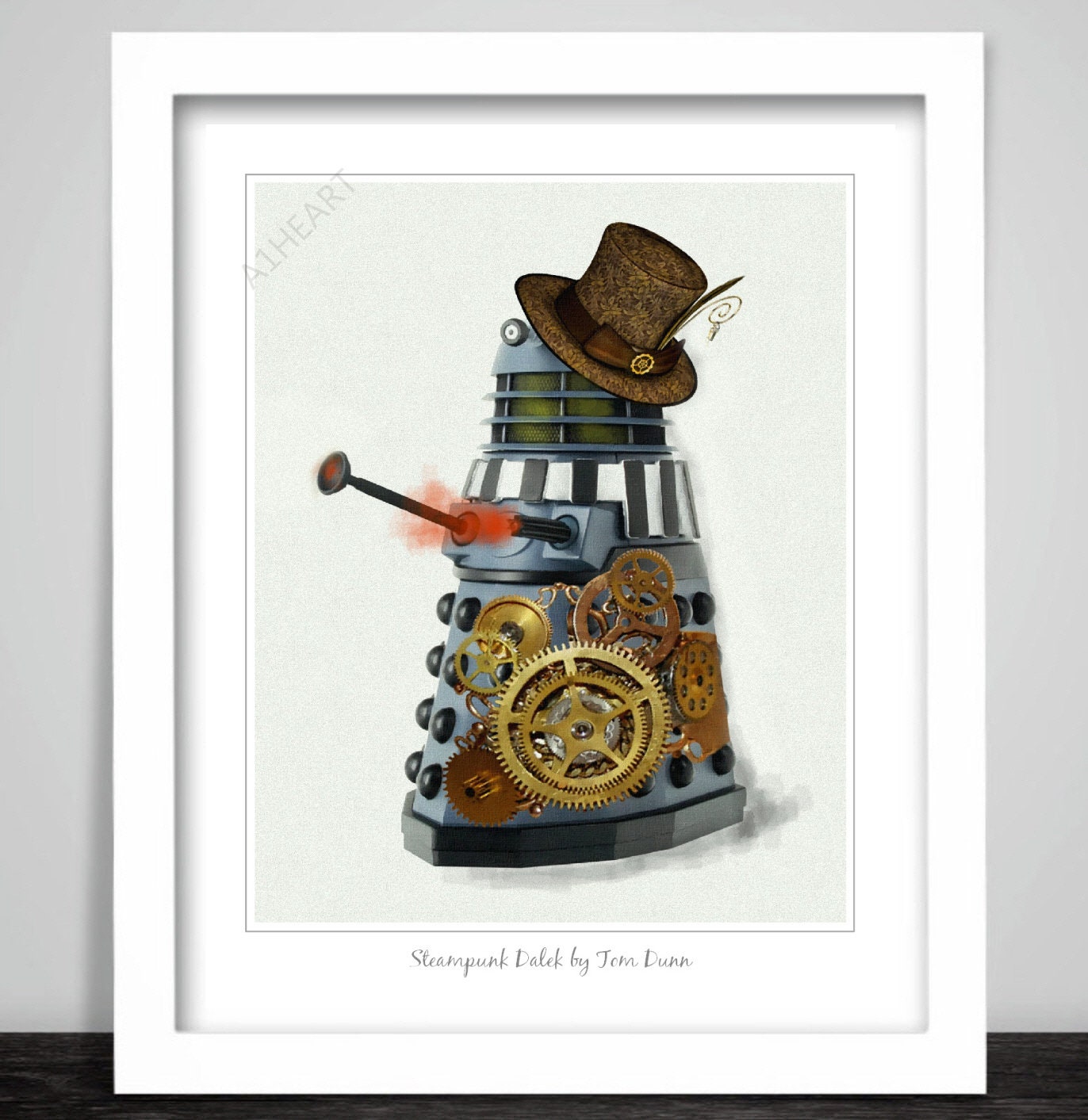The image is a multi-color digital graphic titled "Steampunk Dalek" by Tom Dunn. It features a robot designed in the distinctive steampunk style, adorned with various gold, bronze, and copper gears of different sizes. The Dalek, a recognizable character for Doctor Who fans, sports a brown steampunk top hat and is equipped with a front-mounted laser gun. The robot's single eye is prominently placed at the top, reminiscent of R2D2. The artwork is presented within a series of frames: a thin black frame closest to the image, encased by two white frames of varying thickness, all set against a gray background that forms a border at the top and sides. The piece appears to rest on a black surface, likely a table or countertop. At the very bottom of the image, the title "Steampunk Dalek by Tom Dunn" serves as a clear identifier.